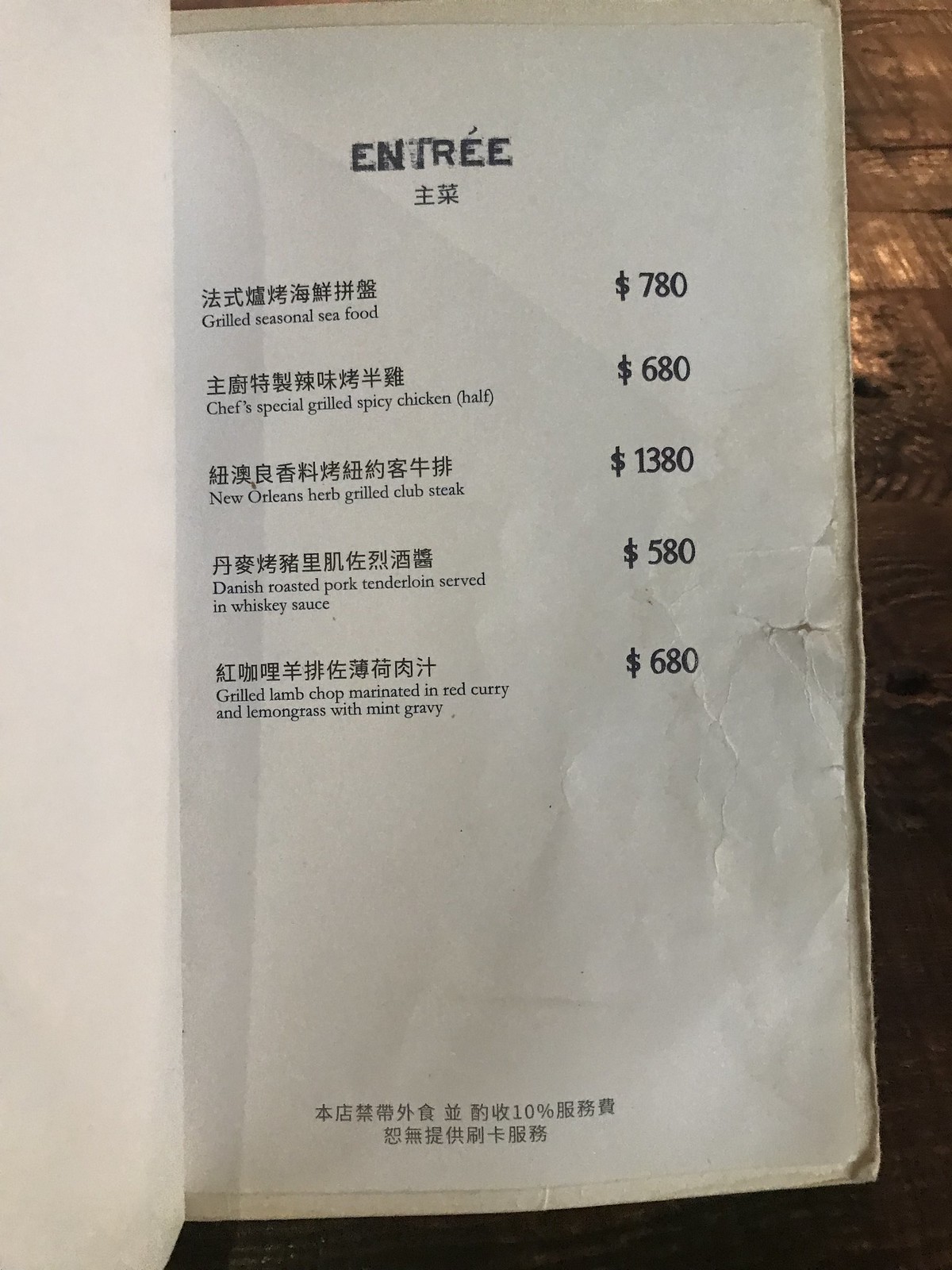The image showcases a menu page set against an ivory-colored piece of cardboard, partially turned over, revealing its connection to the book binding. The background features a rustic wooden table with horizontal strips of lumber, varying in color from dark brown at the bottom to lighter shades as they ascend.

At the top of the menu, the word "Entrée" is prominently displayed in black letters, complete with an accent over the second 'e.' Beneath this, two Chinese characters indicate that the menu is from a Chinese restaurant. The items listed are presented first in Chinese, followed by an English translation and the prices:

1. Grilled Seasonal Seafood - $780
2. Chef's Special Grilled Spicy Chicken Half - $680
3. New Orleans Herb Grilled Club Steak - $1,380
4. Danish Roasted Pork Tenderloin Served in Whiskey Sauce - $580
5. Grilled Lamb Chop Marinated in Red Curry and Lemongrass with Mint Gravy - $680

At the bottom of the page, additional Chinese text is visible, though it does not have an accompanying English translation.